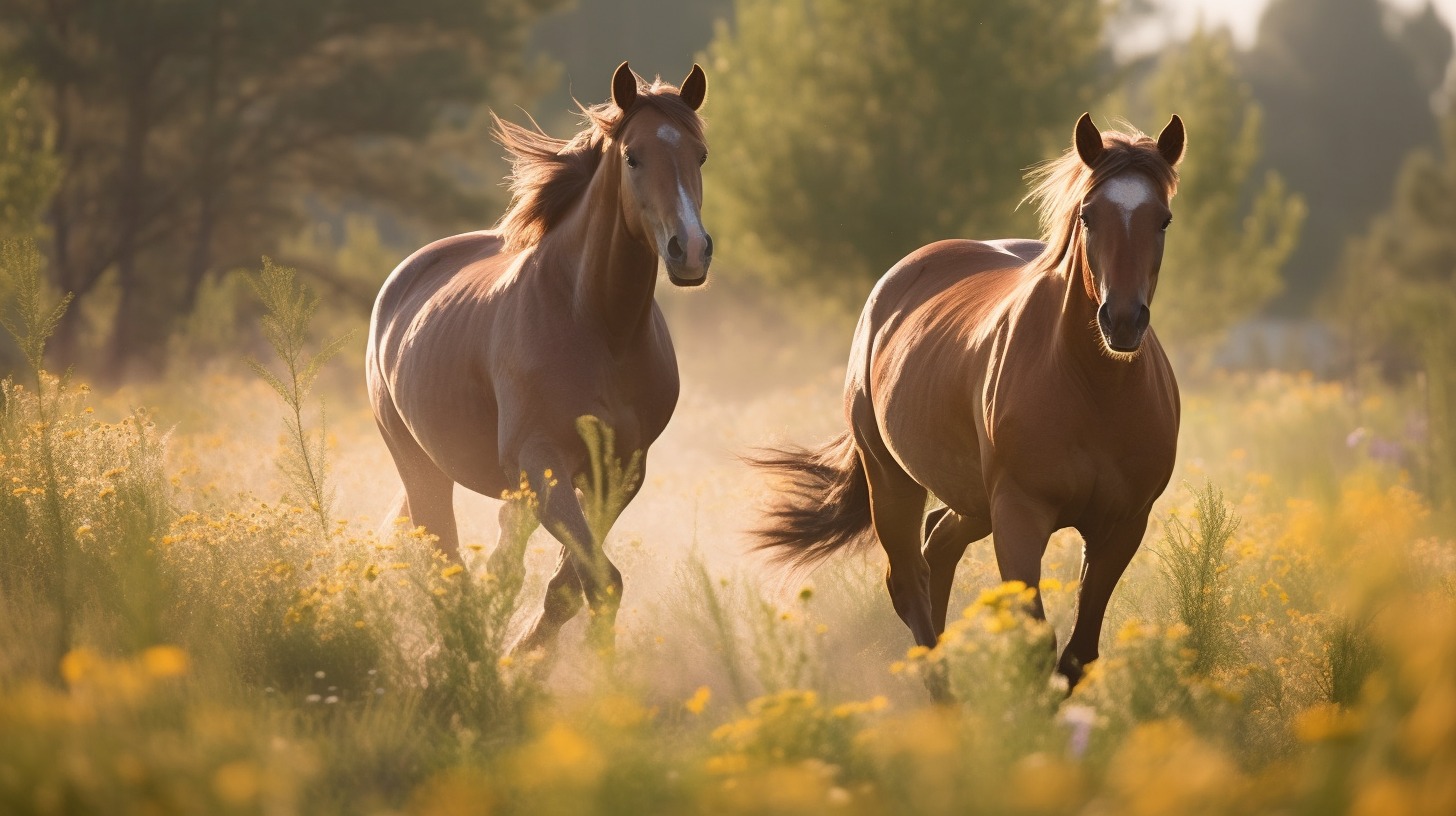The image depicts two wild horses galloping through a vibrant field of tall yellow flowers and green weeds. The horses are light brown with distinctive white patches: one has a large white spot on its forehead, and the other has white on its nose. Their manes are flowing in the wind, with one horse having a lighter mane and the other a darker one. They are running side by side, facing the camera, with the horse on the right's head slightly turned forward and the one on the left's head turned slightly to the right. Behind them, the sun shines brightly, casting a blur over the green trees and creating shadows on the front of the horses and to the right of the image. The sunlight adds a warm glow, highlighting the tans, browns, whites, and the vivid yellows of the flowers. The ground behind them shows a faint trace of dust or smoke, emphasizing their swift movement and free spirit. The overall scene is sunny and full of natural beauty.